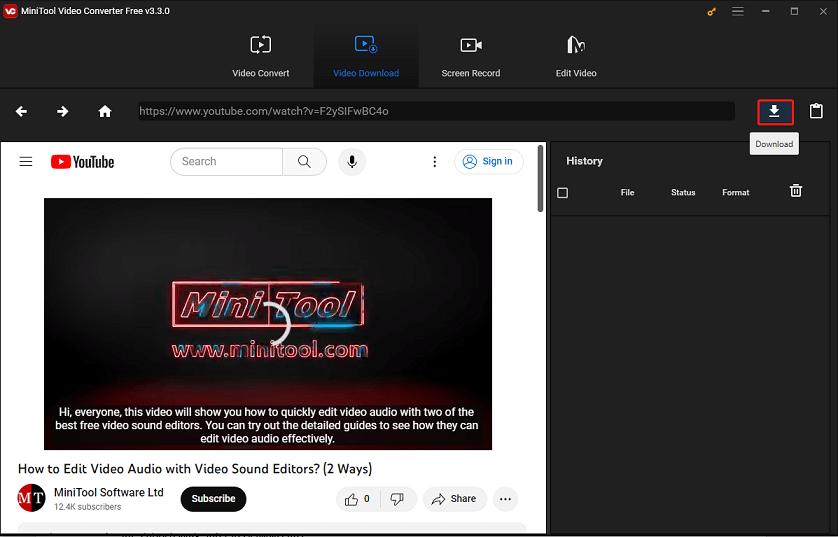The image predominantly features a dark background. In the top left corner, it displays "MiniTool Video Converter Free, version 3.3.0." Centered near the top are four tabs labeled "Video Convert," "Video Download," "Screen Record," and "Edit Video." Beneath these tabs, there are navigation icons: a white arrow pointing left, a white arrow pointing right, and a home symbol. Adjacent to these icons is a search bar containing a web address, specifically "youtube.com/watch" followed by a unique identifier.

Next to the search bar, a white arrow pointing downward, encased in a red square, denotes a download option. Directly below this is a gray "Download" button, and to its right, a clipboard icon. Further down, there is a white rectangular section displaying what appears to be a YouTube interface. The video title shown is "How to Edit Video Audio with Video Sound Editors Two Ways," published by MiniTool Software LTD, which has 12,400 subscribers. The video's opening text reads: "Hi everyone, this video will show you how to quickly edit video audio with two of the best free video sound editors. You can try out the detailed guides to see how they can edit video effectively."

On the right side of the image, the sidebar includes headings such as "History," "File Status," "Format," and an icon of a trash can.